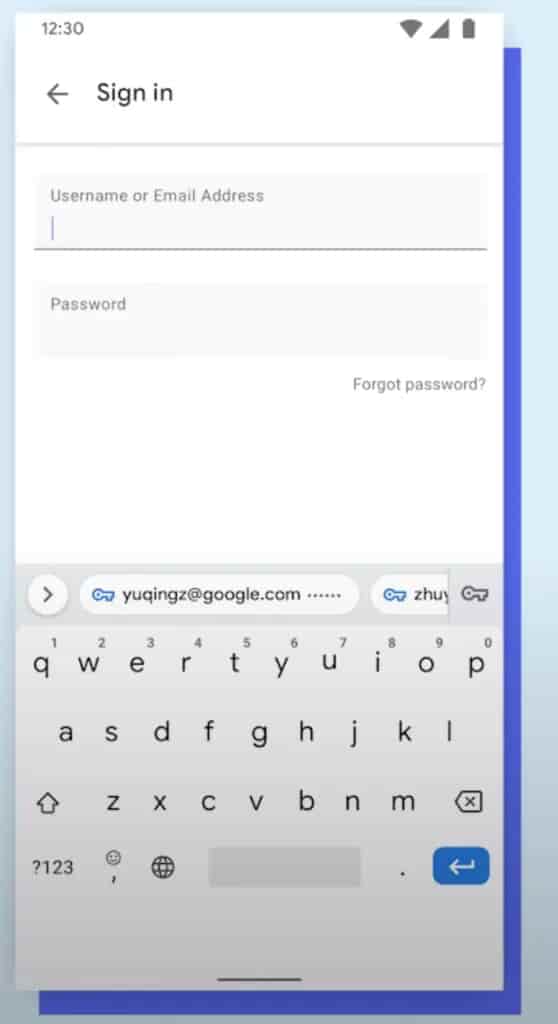The image showcases a digital interface with a minimalist and efficient design. The background features a gradient in shades of blue. Centered within the blue background is a white rectangular area, visually highlighted by a dark blue shadowed border on the right-hand side.

In the top-right corner of the white rectangle, a digital clock displays "12:30" in black text. Adjacent to it, on the very right edge, are icons indicating full Wi-Fi signal, full cellular signal, and a fully charged battery.

On the next line down, to the left, there's a back-arrow icon pointing to the left, followed by the text "Sign In." Below this line, a thin gray bar stretches across the width of the white rectangle. Beneath the bar is a field for entering a username or email address, currently empty, followed by another field for entering a password, also empty.

At the bottom right of these input fields, the text "Forgot Password?" appears in gray, accompanied by a question mark.

Below the input fields, a virtual keyboard occupies the lower portion of the screen. The keyboard layout is QWERTY, with keys in a contrasting gray and black color scheme. The top row includes numbers one through nine, with the zero placed above the "P" key. Additional function keys appear at the bottom, including a question mark, a numerical toggle key (labeled "123"), emoji access, web key, a period key, and a prominent blue "Enter" key. A unique white circular button with an open-arrow icon is positioned alongside a blue key labeled "yougookingsatgoogle.com" and another blue key with the text "ZHUY."

At the very bottom of the interface, a gray slider control is visible, offering additional interaction options.

The overall design is functional, user-friendly, and uncluttered, clearly setting the stage for user authentication.